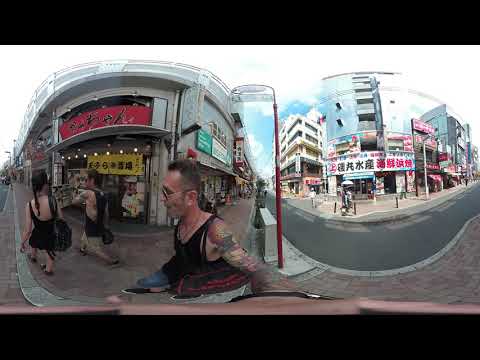The image is a photographic scene set outdoors on a bustling city street during the daytime, captured with a wide-angle lens that distorts the view. The central character is a Caucasian man with a buzz cut, dressed in a black tank top, aviator sunglasses, and blue jeans, showcasing a sleeve of tattoos on his left arm. He appears to be taking a selfie with a camera held downwards. Directly behind him, two individuals of Asian descent are walking. One woman, wearing a short black dress and carrying a backpack, is followed by another individual who resembles the tattooed man in attire—a black tank top and khaki shorts, also adorned with tattoos. The street is lined with various buildings, including a one-story shop featuring prominent yellow and red signs with Asian characters, and taller buildings, four and five stories high, displaying additional Asian signage. The gray street has white markings, and the sky above is filled with white clouds. The image composition includes a black header and footer, framing the scene within rounded shapes, and there are noticeable streetlights in the background.